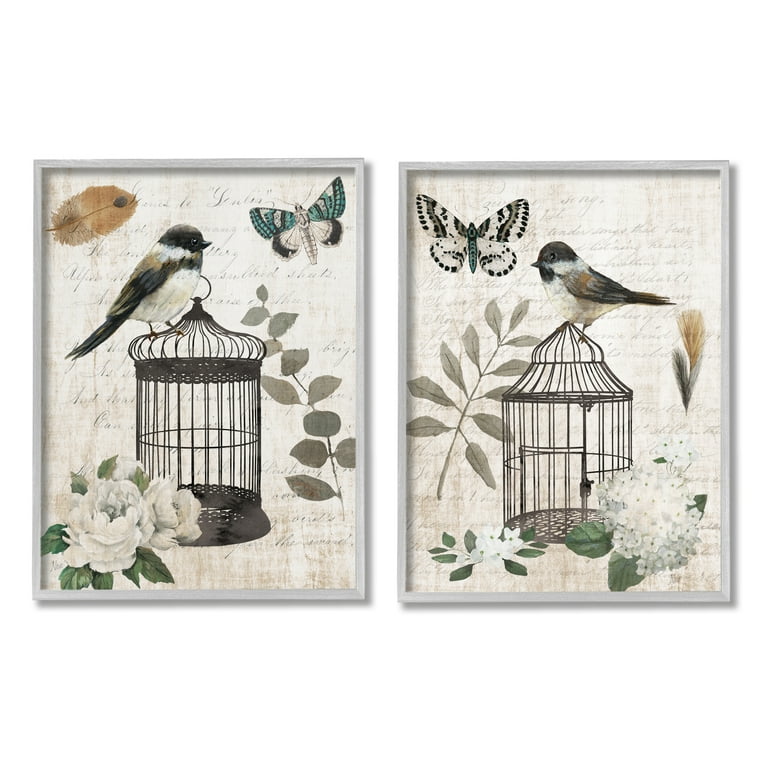The artwork consists of two side-by-side images each depicting a bird standing on a birdcage, rendered in a photo-realistic style. The birds, likely of the same species, have distinct features with black heads, black feathers, and white bellies. The bird on the left image stands on the left side of its dome-shaped birdcage, whereas the bird on the right image is perched on the right side of a more triangular dome-like cage, both considerably larger than the birds themselves. Surrounding the central figures, each artwork is embellished with natural elements such as pressed butterflies, flowers, leaves, and petals, arranged differently in each image. The backgrounds of both images are filled with faded, handwritten script, evoking the appearance of old letters or a sketchbook. The images, which seem like a collage of various art forms including watercolor and photorealistic elements, feature blue, white, and black butterflies and create a harmonious yet varied visual narrative.